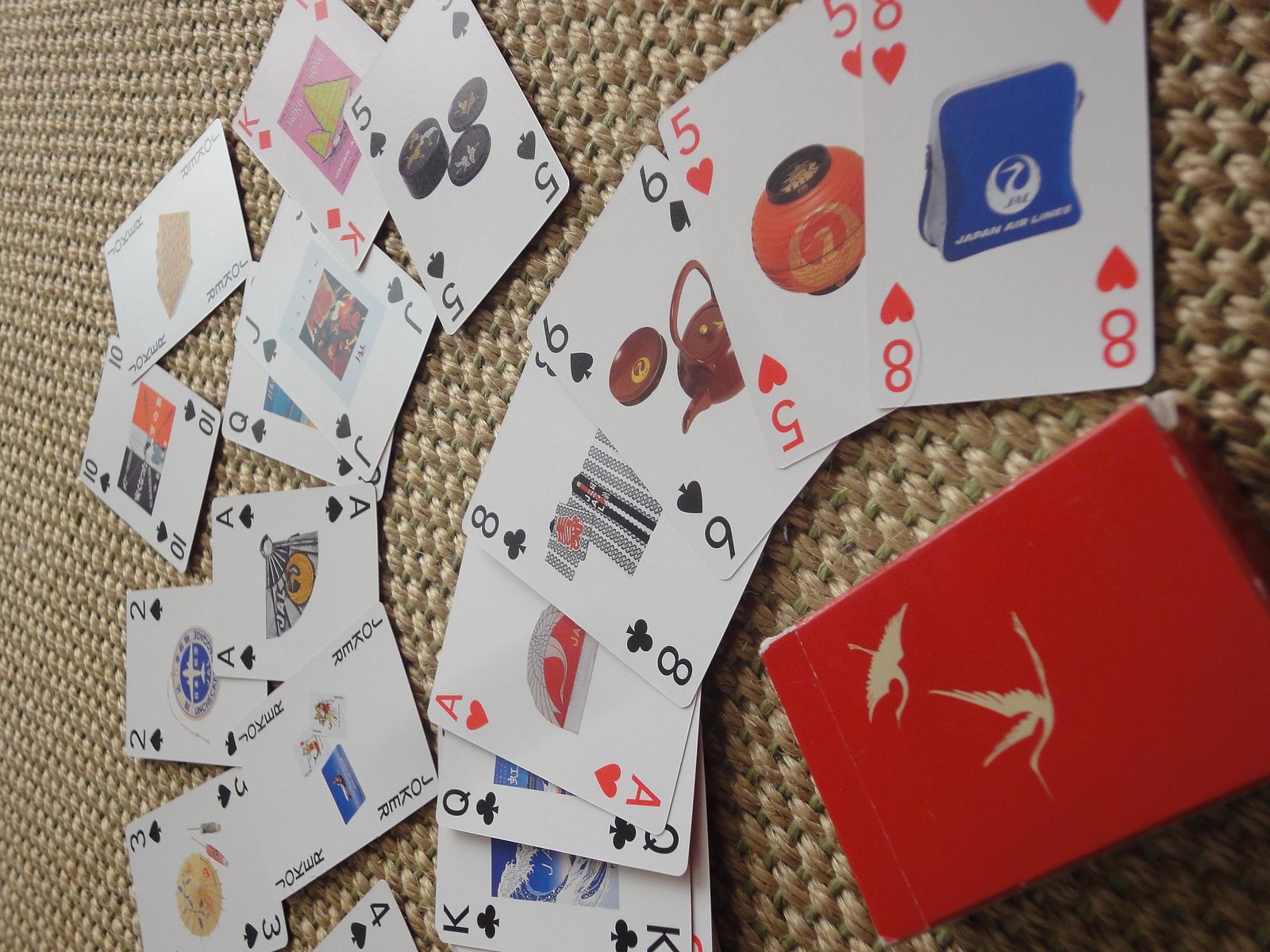This image showcases a unique set of playing cards, each card bearing traditional poker markings—such as the King of Clubs, Queen of Clubs, Ace of Hearts, Eight of Clubs, Six of Spades, Five of Hearts, Eight of Hearts, and more—exquisitely arranged in a deliberate pattern, all face-up. Notably, there are two Jokers included in the spread. What's particularly striking about this set is the intricate Japanese-themed artwork adorning the center of each card. For instance, the Eight of Hearts features an image of a blue and gray bag emblazoned with "Japan Airlines." Another card displays a teapot with matching teacups, while yet another features a traditional Japanese fan. One card is decorated with what appear to be poker chips, and another boasts an image of a kimono shirt. Additionally, a prominent red booklet with gold-embossed illustrations of flying birds can be seen. Each card thus combines elements of classic playing card design with vibrant, culturally evocative illustrations, creating a visually rich and captivating scene.